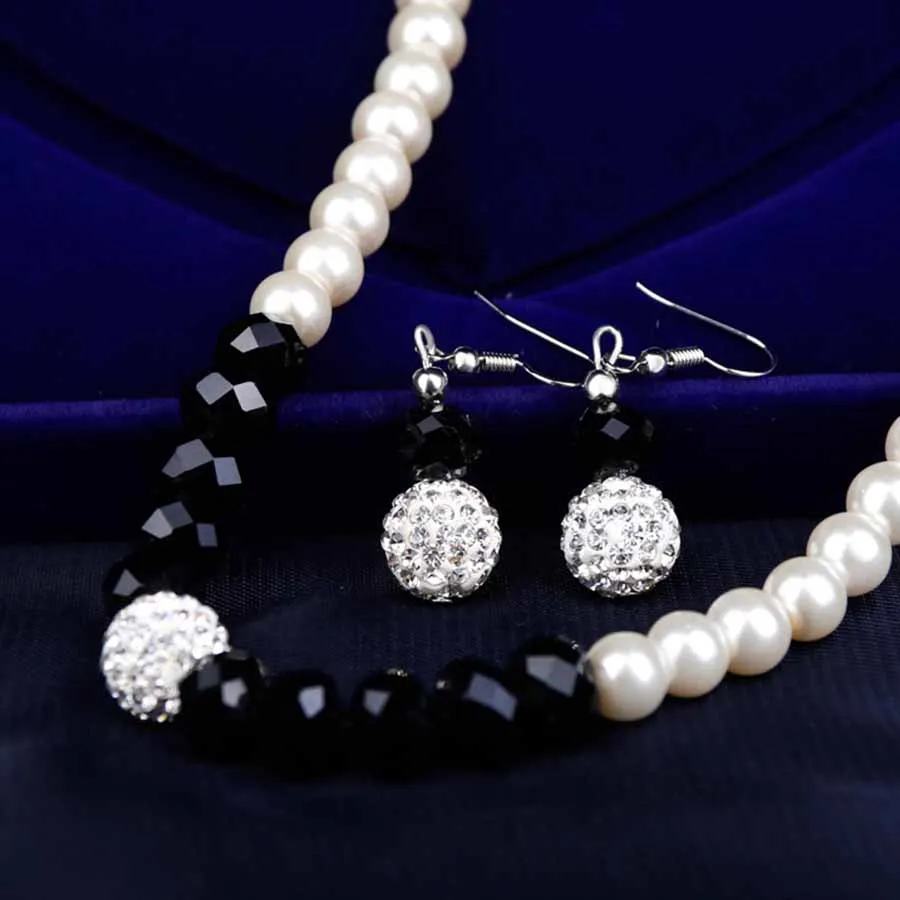The image showcases an elegant set of jewelry against a rich, dark blue velvet background, resembling the interior of a luxury jewelry case. A statement necklace, draped gracefully, features a series of lustrous white pearls linked together, transitioning into sleek black hexagonal beads. At the center, the necklace boasts a dazzling diamond-encrusted sphere. From this focal point, another sequence of black beads and white pearls continues, though the clasp and the full length of the necklace are not visible. Accompanying the necklace are a pair of matching earrings, positioned within the necklace's loop. The earrings highlight round, diamond-encrusted spheres identical to the centerpiece of the necklace, each adorned with a single black bead. They feature hook-style, silver clasps, designed for pierced ears. This harmonious arrangement emphasizes the meticulous craftsmanship and design cohesion between the necklace and the earrings.